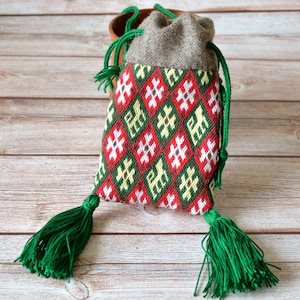The image displays a handmade, medium-sized bag with a festive, Christmas-like design. The bag features a prominent diamond checkered pattern in red, green, and white. The red squares contain intricate snowflake-like or granny square shapes, while the green ones display similar patterns along with small lion designs. The bag is topped with a soft, gray fleece material and has green paracord-type drawstrings for handles. Green tassels are attached to each bottom corner of the bag. The setting for the photo is a rustic, wooden backdrop with visible planks that enhance the handcrafted feel of the scene.